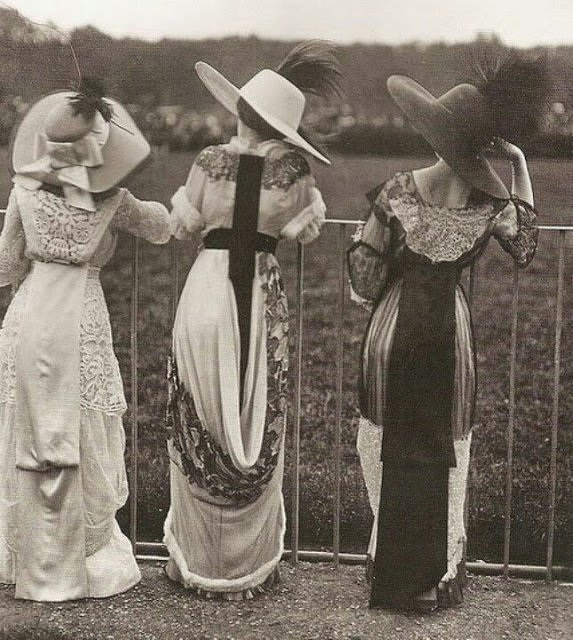This vintage, square-shaped black-and-white photograph, tinged with a hint of sepia, captures three women from the early 1900s standing side by side. All three women are facing away from the camera, leaning their arms on a tall metal fence made up of bars. Each woman is adorned in a floor-length Edwardian dress and a large, wide-brim hat topped with feather plumes.

The woman on the far left dons a dress with Queen Anne's lace-shaped patterns and a large sun hat with a ribbon and a black feather. Her dress is completely white. The woman in the center wears a white dress with black garnishings, including a belt around her waist and a black stripe running the length of her dress at the back. Her wide-brim hat is also white with a black feather. The woman on the right is dressed mostly in black, with her dress extending to her feet. Her dark brown hat features a matching black feather.

They stand on a gravel pathway, gazing out over a well-maintained lawn that stretches into the distance, ultimately merging with a horizon filled with multiple trees.